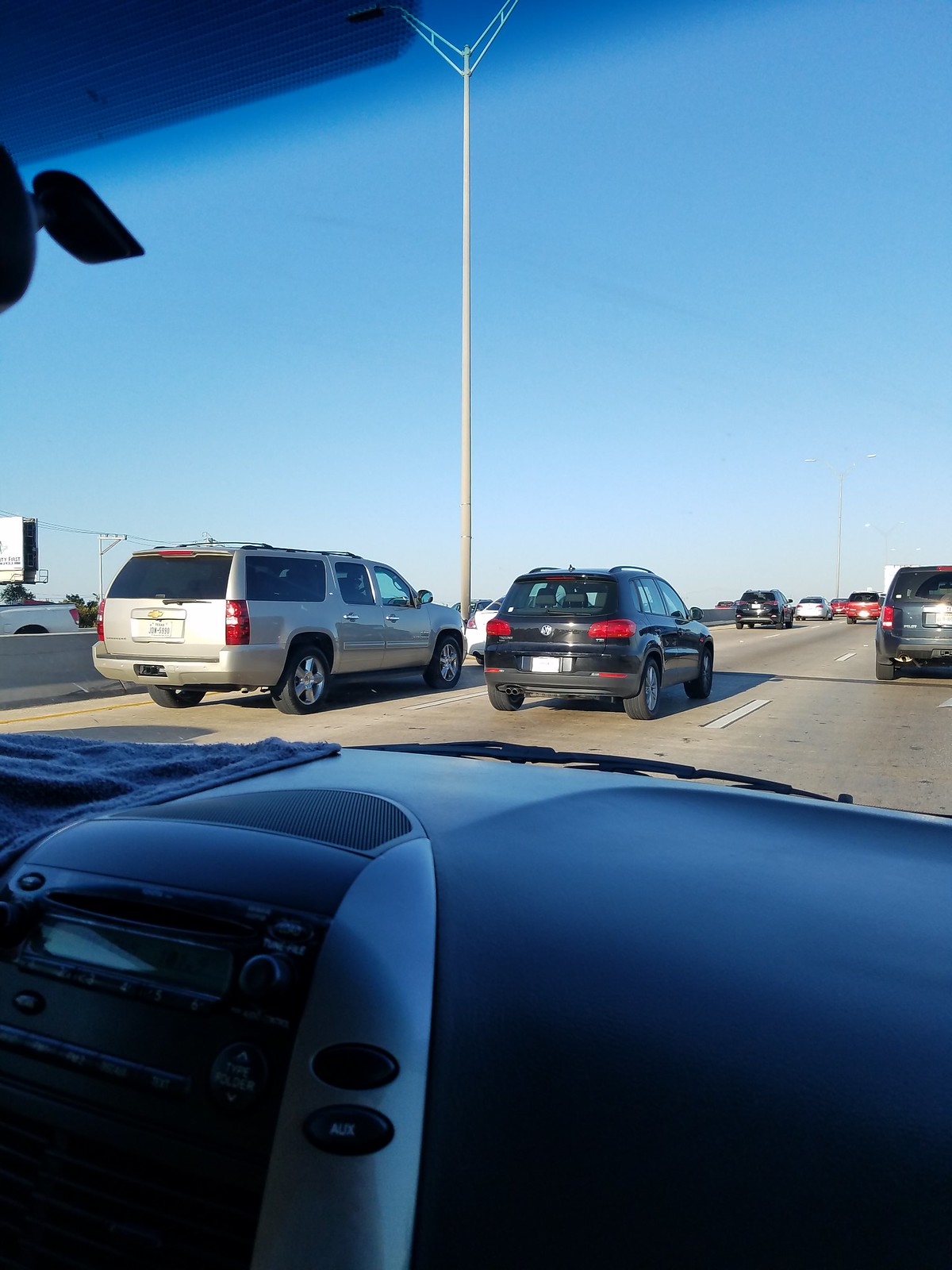This image appears to be a photograph taken from the passenger seat of a parked vehicle, likely on the roof of a parking garage or a flat parking lot. The dashboard, noticeable for its black interior and partial view of the radio, dominates the lower half of the frame, with a piece of cloth draped over part of it. Through the windshield, several rows of parked cars extend into the distance under a blue and cloudless sky. Closest to the vehicle are two parked cars on the left and center of the next row: a silver-gold large SUV and a black compact car. The following row, visible further back, includes another parked car to the right and additional scattered vehicles across the lot. A light pole is also visible among the cars. The overall scene appears to capture a bright, sunny day as viewed from the stationary car.